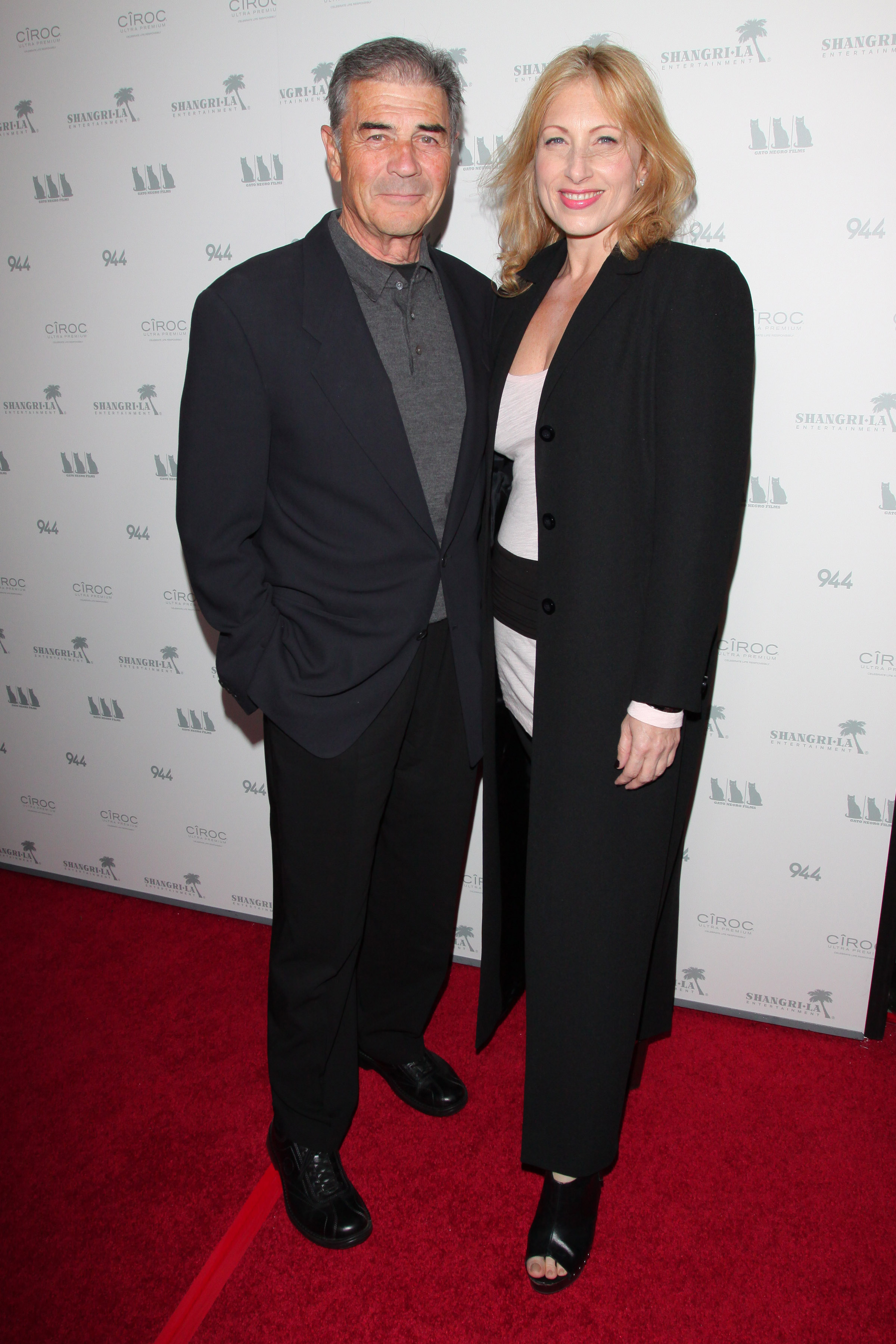In this photograph, a couple is captured at a red carpet event, standing side by side. The man on the left, who appears to be a famous actor though his identity is not recalled, has dark hair with some silver strands and dark eyebrows. He is dressed in a black suit paired with a dark gray polo shirt, black trousers, and black shoes. His hands are casually placed in his pockets, and he is smiling softly at the camera. The woman on the right, presumed to be his wife, has long blonde hair and is also smiling. She is wearing a lengthy black coat resembling a suit jacket that extends to her ankles, a white blouse, and black open-toed shoes. The couple stands in front of a backdrop adorned with various sponsor logos, including "Shangri-La," "944," and "CÎROC," with images such as palm trees scattered throughout the background.